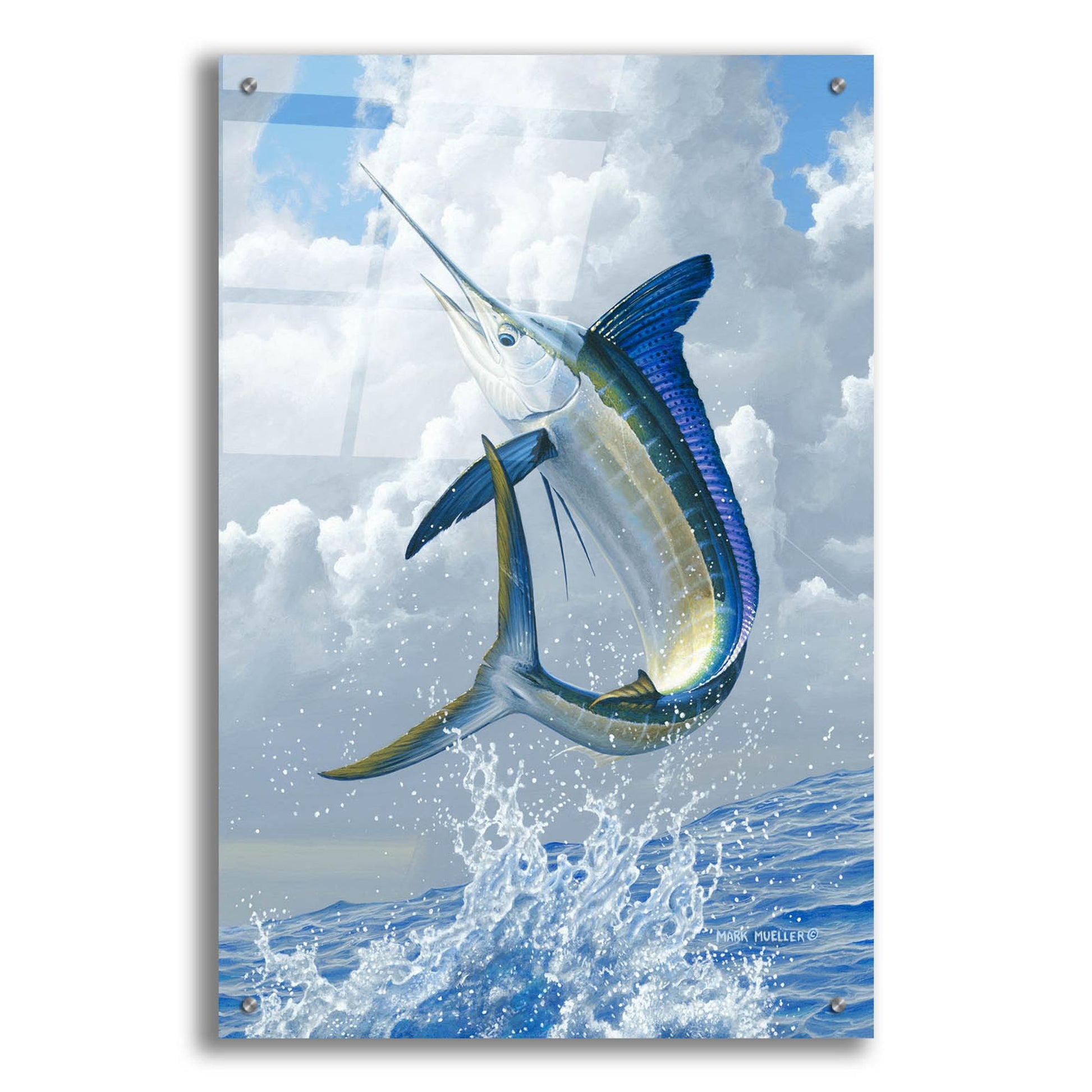This detailed painting captures a vibrant scene of a marlin or swordfish, portrayed in a realistic yet fantastical style, dramatically leaping out of tumultuous blue waters. The fish's sleek body boasts a striking color scheme of deep blue fins and a shimmering silver belly, with its pointed nose directed towards the upper left corner of the image. Set against a dynamic backdrop, the sky is filled with billowing white clouds, allowing glimpses of bright blue to peek through, enhancing the overall luminosity and movement of the scene. The painting, taller than it is wide, reminiscent of magazine dimensions, exudes a sense of motion and energy, emphasized by the water's splash as the fish breaches the surface. The bottom right-hand corner of the artwork bears the signature "Mark Mueller" followed by a copyright symbol, confirming the piece's authenticity and ownership.